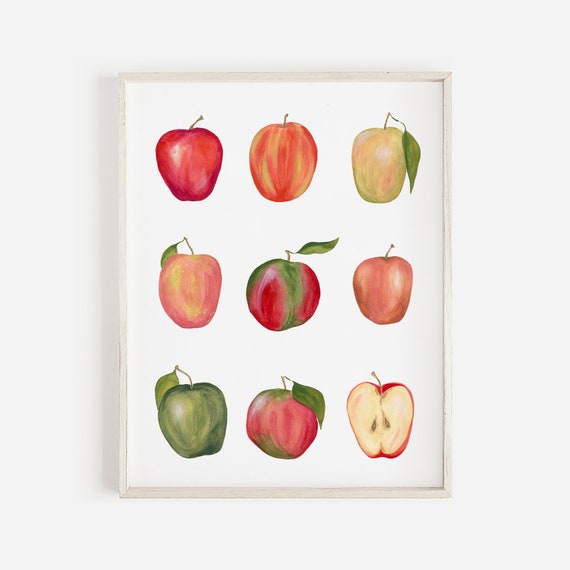This is an image depicting a rectangular piece of artwork that appears to be hanging on a white wall, framed in a simple, lightly-colored wooden frame. The artwork itself has a white background and features nine realistically painted apples, arranged in a grid pattern of three rows by three columns. Each apple is distinct in color and detail, suggesting a variety of types and artistic techniques such as colored pencils or watercolor.

Starting from the top row, the upper left apple is a classic red variety. In the upper middle position, there's an apple with blended red and yellow hues, resembling a rounder variety. The upper right apple is vibrant green with a single leaf attached to its stem. 

Moving to the middle row, the apple on the left slightly resembles a peach, complete with a leaf hanging to the left of the stem. The central apple is primarily red with a green stripe, showcasing a leaf that appears to be fluttering to the right. On the far right of this row is a pale pink or light peach-colored apple.

In the bottom row, the apple on the left is very dark green with a leaf extending to the left. The central apple in this row is predominantly red with green at both the top and bottom, complemented by a leaf on the right. Lastly, the bottom right apple is presented as a cross-section, revealing the white flesh and seeds inside, with its red skin still visible around the edges.

The entire piece delivers a cohesive artistic study of different apple varieties through a meticulous and colorful representation.